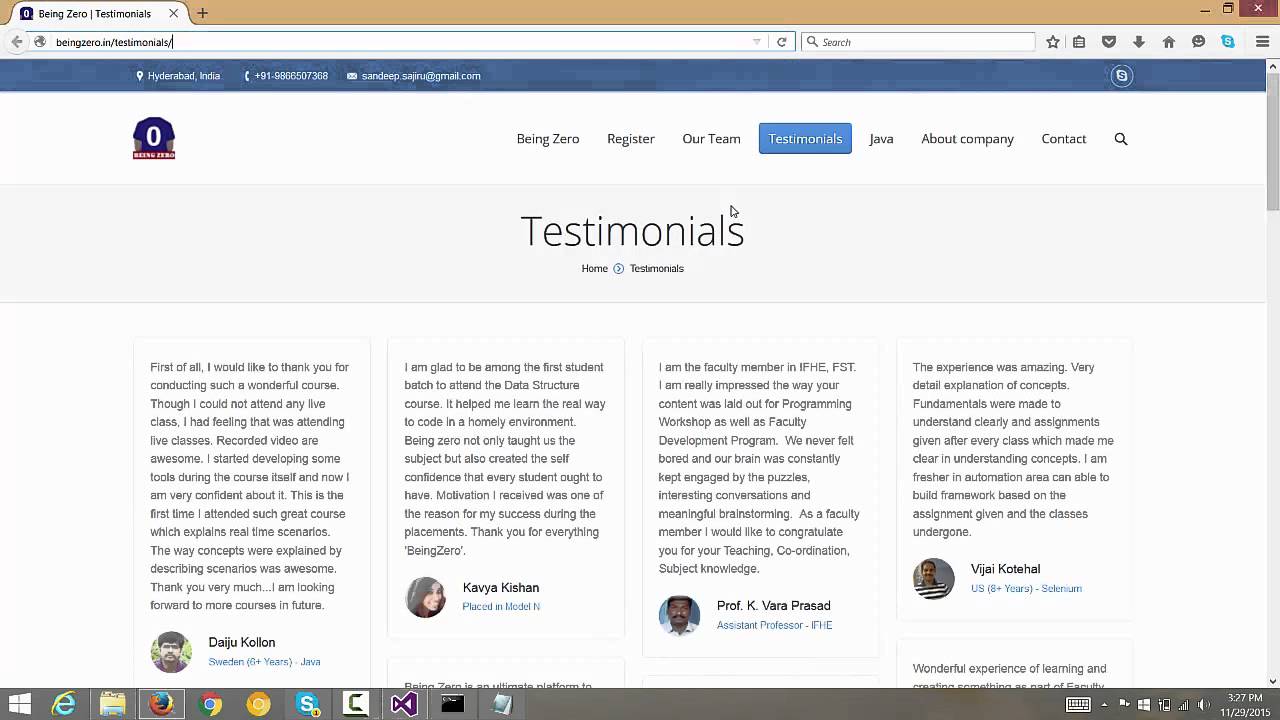The screenshot captures a rectangular section of a testimonial webpage, likely taken on a desktop or laptop. The webpage primarily features a clean, white background with dark gray text. At the top center of the image, within the upper 25%, the word "Testimonials" is prominently displayed in a larger font. Above this heading, a horizontally laid-out menu offers various options in black text. One of the options, "Testimonials," is centrally located and situated between "Our Team" and "Jobs." This menu item is highlighted with a dark blue rectangular background and white text, resembling a clickable button.

Beneath the main "Testimonials" heading, four distinct reviews from different users are displayed. Each review consists of a paragraph of feedback about the website and its products. Accompanying these written testimonials are circular profile pictures of the reviewers, each captioned with the user's name in bold black text. Below each name, additional details are provided in a light blue font.

The webpage is bordered by a dark blue strip at the top and a dark gray strip at the bottom. The bottom strip also shows the user's computer controls and various icons, including Internet Explorer, Mozilla Firefox, and Google Chrome.